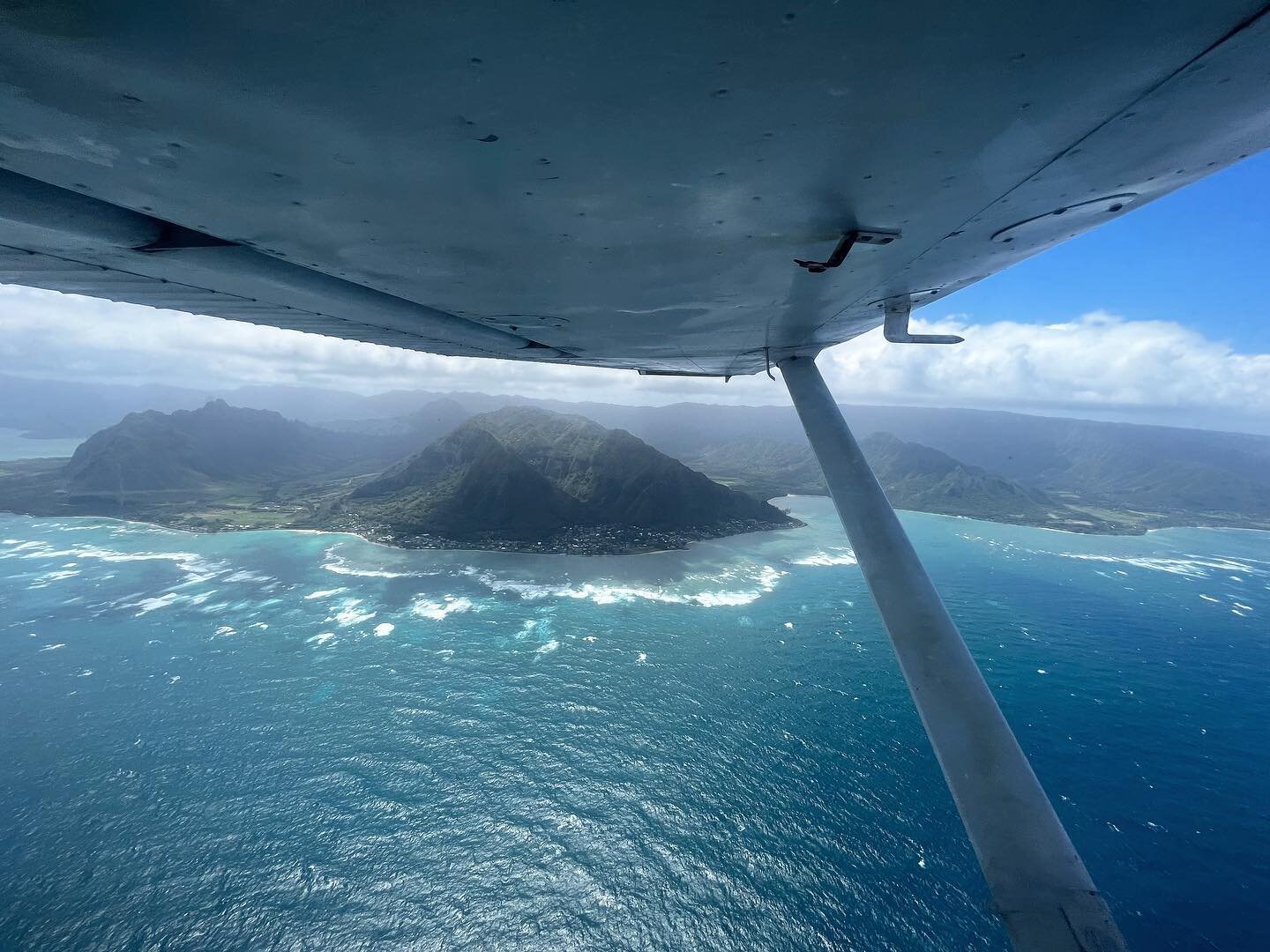Captured from high above, this photograph showcases a serene and expansive ocean view, likely taken from underneath the wing of an airplane. The image prominently features a calm, blue-green sea with waves gently breaking against an island's rocky shore. The island itself is mountainous, with lush green slopes suggesting abundant vegetation. Scattered across the island are small indistinct specks, hinting at buildings or cars in what appears to be a small city. The sky overhead is a picturesque mix of vivid blue and a bank of white and grayish clouds on the horizon. The airplane’s white wing and a support bar are visible in the foreground, grounding the viewer's perspective as they gaze out over the tranquil body of water and rugged island terrain below.